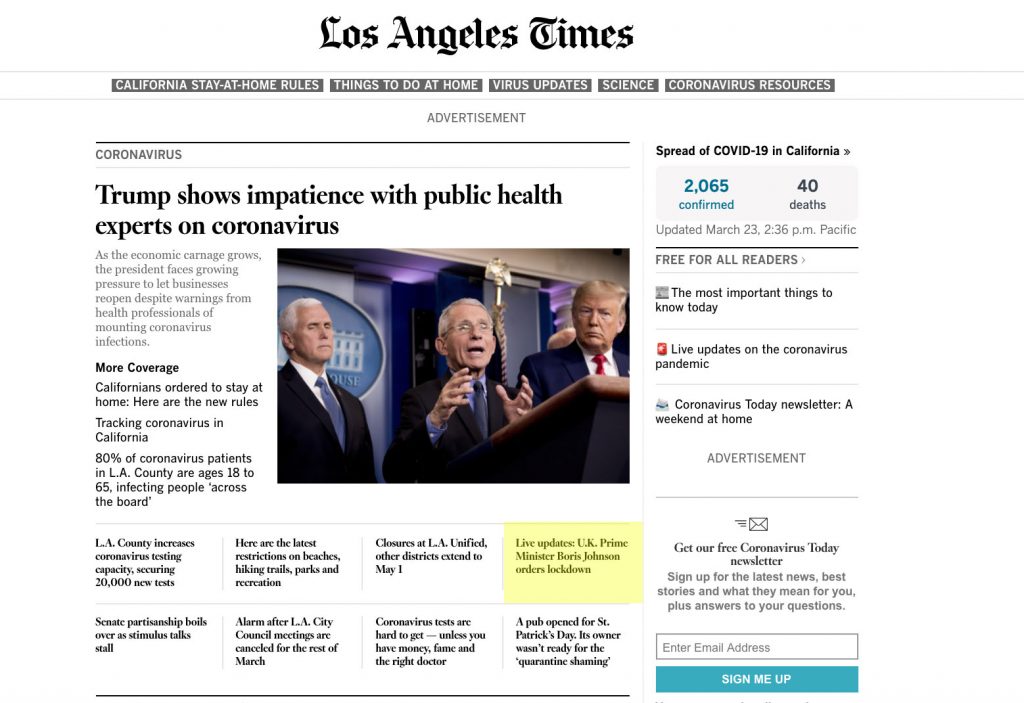**Image Caption:**

In this poignant image featured in the Los Angeles Times, President Donald Trump stands in front of an audience, visibly displaying his impatience with public health experts regarding the coronavirus pandemic. The picture captures a moment during a press briefing, where an older man is positioned at a podium, likely addressing the pressing issue of COVID-19 amidst a backdrop of economic devastation. As the toll on the economy intensifies, Trump faces escalating pressure to allow businesses to reopen, despite stern warnings from health professionals about escalating infection rates. The accompanying article provides extensive coverage, including new directives for Californians to stay at home, the statistical tracking of coronavirus cases in California, with 80% of LA County patients aged between 18 and 65, and the county's effort to increase testing capacity by securing 20,000 new tests.